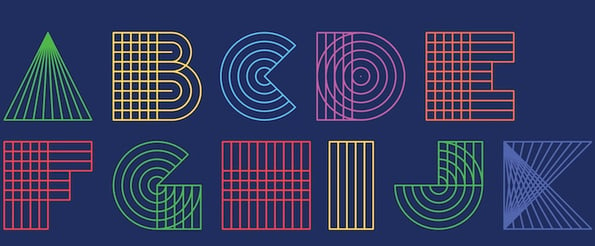The image is a rectangular graphic with a blue-gray background, showcasing the alphabet from A to K in two rows. Each letter is depicted with a unique geometric design characterized by lines, grids, and circles. The letter A appears as a green pyramid with lines emanating from its peak. The B features boxes for its vertical line and semicircles forming the loops, adorned with various interconnecting lines and squares. C resembles a blue Ms. Pac-Man shape. The D presents as a box with an inner circle and lines. E resembles the B design but in orange, and F mirrors this style in red. G combines the Ms. Pac-Man motif with a small green box. The H is a simple box with red horizontal lines, while I is a rectangle with yellow lines. J resembles a backward Ms. Pac-Man with a tiny box included. Finally, K consists of intersecting blue lines forming a diamond-like pattern. The letters are rendered in a palette of light blue, yellow, pink, orange, green, purple, and red, all arranged neatly within the wide, narrow frame.